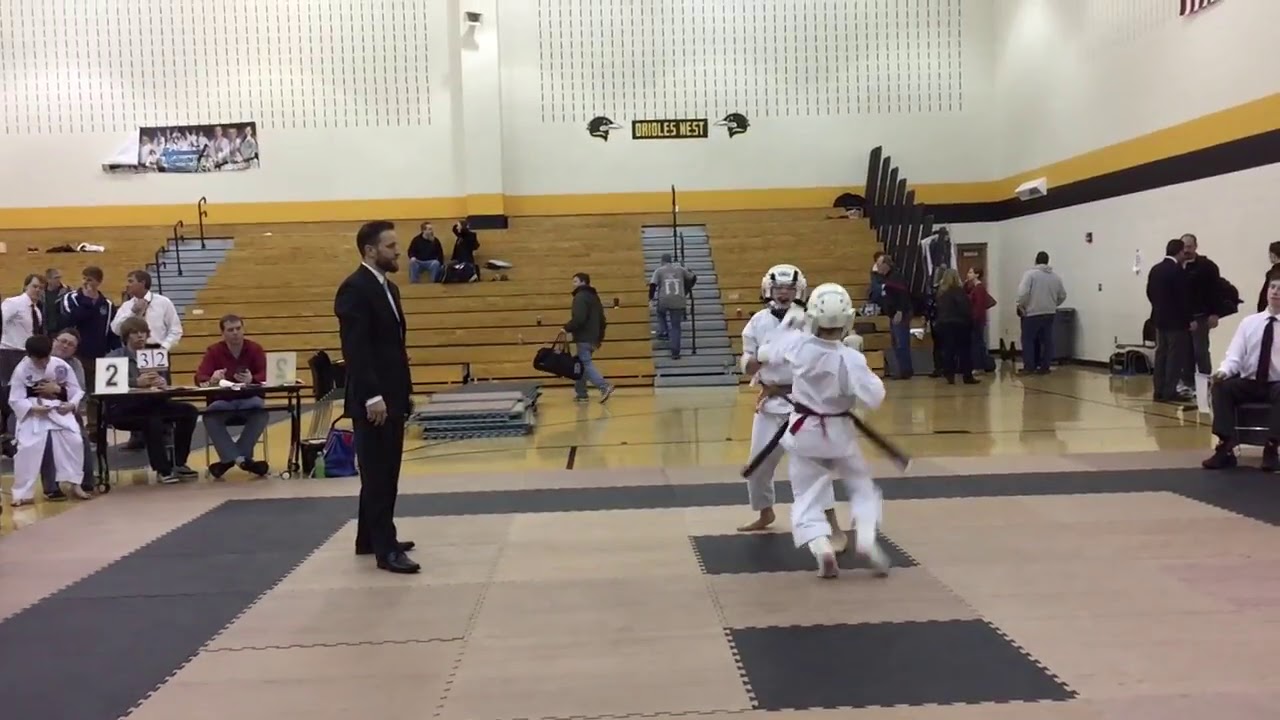This detailed photograph captures the thrilling atmosphere of a martial arts tournament taking place in an indoor gymnasium. In the middle right of the image, two young children dressed in white karate uniforms, each adorned with red and green belts, are intensely sparring while wearing protective white helmets. Overseeing their match is a referee, distinguished in a black suit with a white shirt and tie, who stands attentively between them and another karate student waiting in the background beside a prominent number "2".

Surrounding the sparring area, the gym's floor has a mix of gray and brown hues. The walls are striking with their yellow, black, and white colors, adding vibrancy to the scene. Spectators fill the bleachers and line the walls, some seated and some standing, soaking in the action. To the left, a score table is manned by judges dressed casually in red shirts and blue jeans, capturing the scores as the bout progresses.

Adding a touch of unique character to the venue, a sign proclaims "Orioles West" with two representations of Orioles flanking the text. The overall image is bustling with activity, as people walk around the stands and judges remain focused on ensuring the competition's fairness.